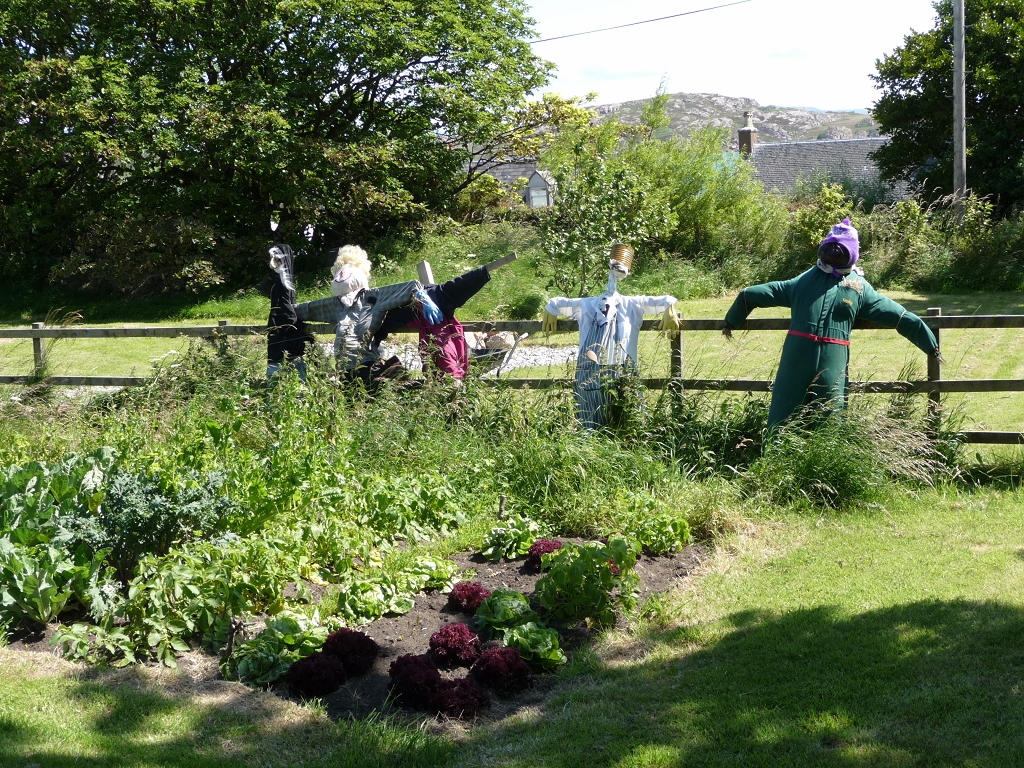In this detailed outdoor photograph, the vibrant blue sky with patches of white clouds serves as the backdrop to a picturesque rural scene. A sprawling mountain range with gray rocky outcrops and grassy patches stretches across the horizon. In the midground, the roof of a house with brownish-gray shingles peeks out, complete with a protruding brick chimney. 

Tall, lush trees in varying shades of green, along with some shorter trees and a telephone pole threading its way through, frame the scene. The landscape's undulating greenery seamlessly transitions into a yard marked off by a robust, waist-high wooden fence. This fence, constructed from thick wood, separates the yard into distinct sections.

In the foreground, a meticulously maintained garden boasts rows of dark maroon plum plants and other vegetables, each row clearly demarcated in the soil. In front of the garden, five distinct scarecrows stand guard, leaning against the wooden fence. These scarecrows are dressed in a variety of outfits: 

1. A thin figure with white hair wearing a black hoodie.
2. A traditional scarecrow head in a plaid shirt with blue dish gloves.
3. A headless scarecrow clad in red bottoms and a black top.
4. A scarecrow with a coffee can head and yellow gloves.
5. The rightmost figure garbed in a green jumpsuit with something purple wrapped around its head.

The entire scene is bathed in sunlight, casting gentle shadows across the yard, enhancing the tranquil, rural atmosphere of this charming countryside tableau.